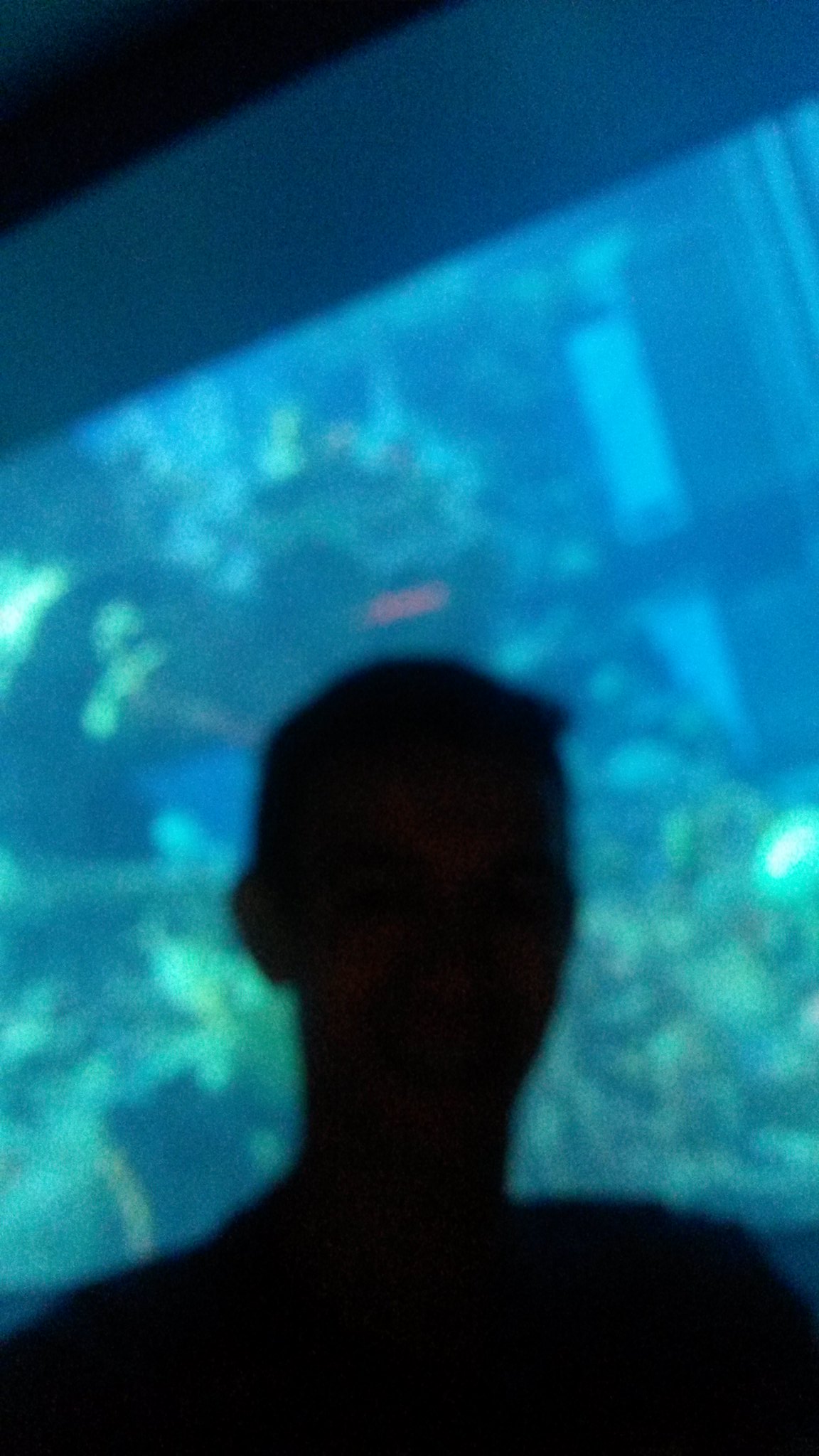The top portion of the image is black, transitioning into a dark blue below it, mimicking the deep sea. Displayed across the screen is an aquarium scene, showcasing an underwater landscape. The aquarium features a variety of corals, including white coral structures scattered on the ground. On the right side, the dark blue merges into a slightly blurry section, indicating a possible out-of-focus element on the screen. In the foreground, at the bottom of the image, stands a person facing the aquarium screen. The individual has short hair, and their head, ear, neck, and shoulders are clearly outlined against the vivid aquatic backdrop.